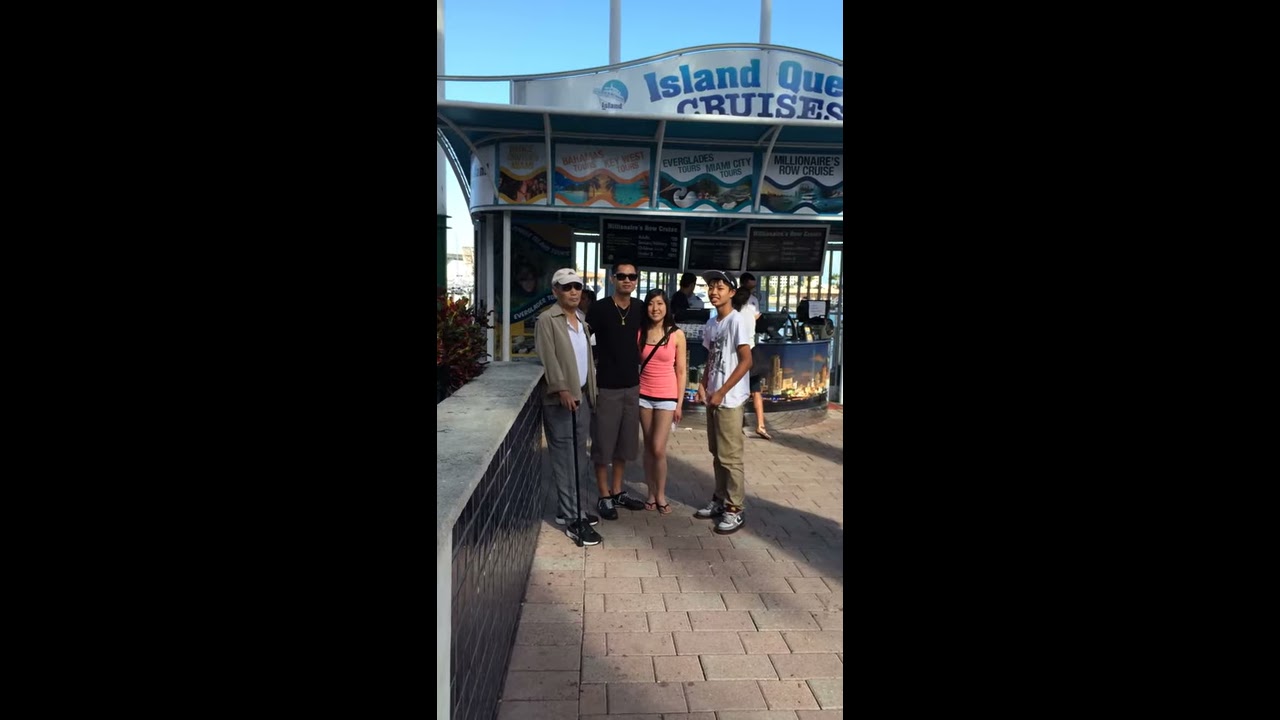In this image, a family of four stands in a row in front of a ticket kiosk for "Island Quest Cruises," which likely offers tours around the Everglades, hinting at a Florida location. The background showcases a cruise or boat adventure setting with a marina feel, featuring paver blocks beneath the group and a small pillar near the kiosk. The ticket kiosk, adorned with blue signage and advertising posters, features three large LCD screens above a rounded counter where people and workers are seen registering for the tours.

The family on the left comprises an older man with a light brown jacket, sunglasses, a light brown baseball cap, a white shirt, gray trousers, and a black cane. Next to him stands a younger man with black hair, clad in a black t-shirt, long black shorts, gray pants, and black sunglasses. Beside him is a woman in a pink (or peach) shirt, white shorts, and sandals. On the far right, there's a young boy wearing a white t-shirt, tan pants, and a black or gray hat. The clear blue sky and slight overhang of the building add to the scene, along with the indistinct menus beneath the "Island Quest Cruises" sign, partially obscured by shadows.